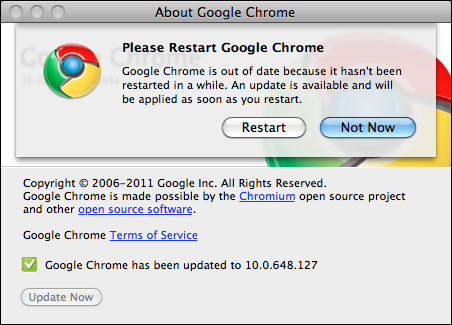The image is a screenshot of the Google Chrome "About" dialogue, displaying various details and hyperlinks. The main dialogue indicates:

1. **Copyright and Acknowledgement**: The text shows "Copyright 2006-2011" and mentions that Chrome is made possible by the [Chromium open-source project](https://www.chromium.org/) and other [open-source software](https://www.google.com/intl/en/chrome/browser/privacy/software.html).
2. **Update Indicator**: A small green checkbox confirms that Google Chrome has been updated to version 10.0.648.127. Below this, there is a grey button labeled "Update Now."

Superimposed on this background is an additional light grey dialogue with a multicolored circular pattern, mirroring Google's color scheme on the left side. The dialogue is titled, "Please restart Google Chrome," and informs the user that "Google Chrome is out of date because it hasn't been restarted in a while. An update is available and will be applied as soon as you restart."

Below this message are two actionable buttons:
- A grey button with black text labeled "Restart"
- A blue button with black text labeled "Not now"

This user-friendly notification prompts the user to restart the browser to apply the latest updates, ensuring optimal performance and security.